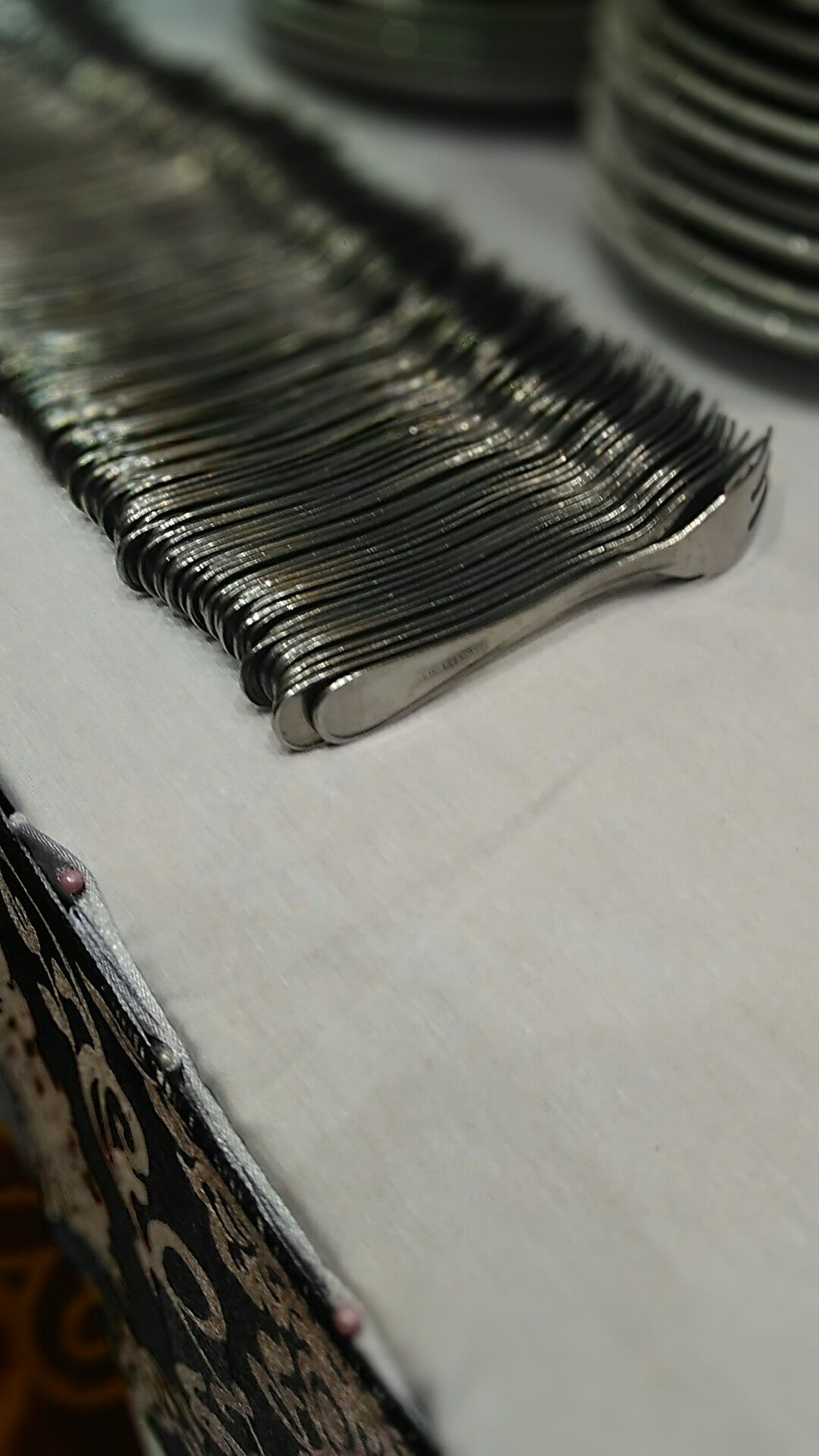This photograph showcases a meticulously arranged, side-on view of a banquet setup. Centered on a white linen tablecloth, which drapes over the side of the bureau revealing a gold and blue intricate design, are hundreds of silver forks lying flat and tightly packed. The forks are stacked on their sides, fanning out diagonally from the middle towards the upper left corner of the image. Each fork boasts the inscription "Cerulean Silver" on the handle and features four tines. The background, slightly blurred, reveals several stacks of ceramic plates in light gray or white, positioned towards the upper right corner. The overall scene presents a sense of organized abundance, with the shiny cutlery forming an almost unbroken line, highlighting the elegance and meticulousness typical of a high-end catering service.